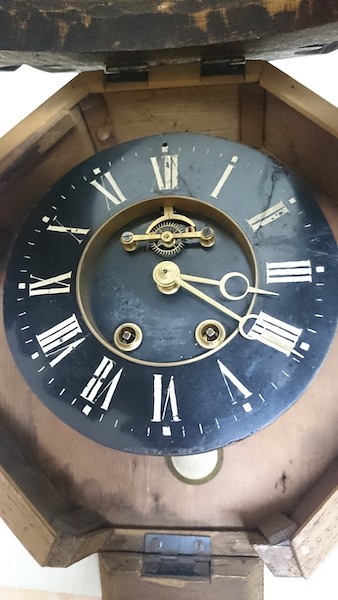This color photograph captures an intricately designed clock housed within a brown wooden octagonal box. The open lid of the box, which is hinged at the top, extends beyond the frame of the image. Visible are signs of water damage inside the wooden interior, adding a rustic, weathered character to the clock's enclosure. The clock face itself is black, adorned with elegant gold Roman numerals that denote the hours. At the top of the clock, just below the 12 o'clock mark, several delicate gears are visible, offering a glimpse into the clock's inner workings. The clock's hands are crafted from gold and feature a circular element just before tapering into pointed tips. The hands are positioned at approximately 3:20. This vertically oriented photograph contains no text or human presence, inviting the viewer to focus solely on the craftsmanship and details of the clock and its encasement.